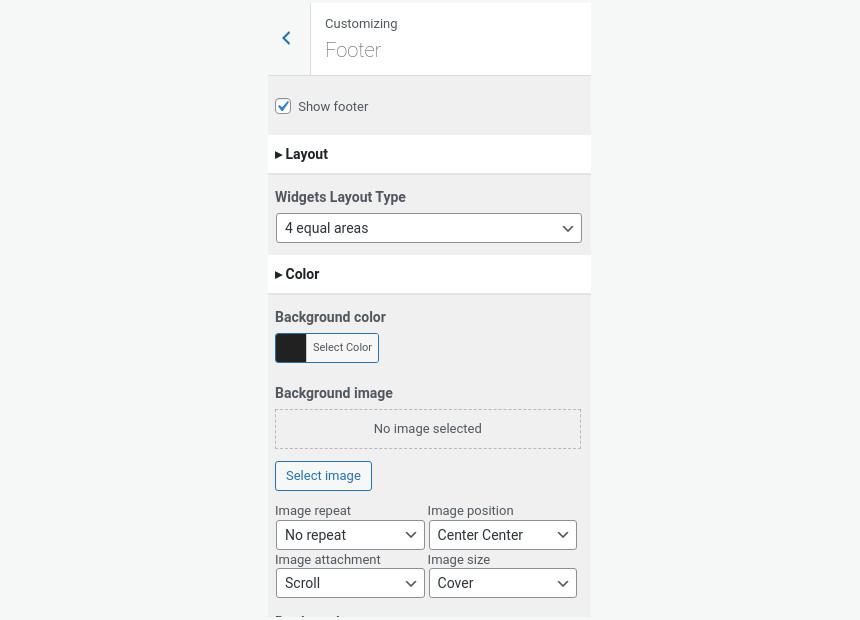The image features a user interface with various customizable options primarily set against a pale gray background. At the top, there is a white rectangular section with black text. The word "Customizing" is prominently displayed in bold font, while "Footer" is rendered in a larger but less bold font. Both "C" and "F" are capitalized. To the left of these words, there's a small blue arrow pointing left.

Below this section, there's a gray rectangle with black text that reads "Show Footer." Adjacent to the "S" in "Show" is a white square containing a blue checkmark. Proceeding downwards, another gray rectangle presents the word "Layout," flanked by a black triangle pointing right next to the "L."

Further down, the text "Widgets Layout Type" follows, with the "W," "L," and "T" capitalized. Below this is a dropdown menu set to "Numerical for equal areas." Finally, at the bottom, there's a white rectangular area containing the word "Color" in bold black text, accompanied by a right-facing arrow next to the "C."